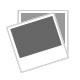This image features a vintage, metal lunchbox with a black outline and handle, resting on a white surface against a white stucco wall. Dominating the front of the lunchbox is a detailed image of a man with curly brown hair and a serious expression, identified as "The Fall Guy." He wears a multicolored leather jacket in greens, blues, and yellows, with his right hand gripping an orange glove and his left hand holding a blue helmet. The upper right corner of the lunchbox showcases the title "The Fall Guy" in blue text. In the background, shades of red, orange, and yellow evoke the appearance of flames, enhancing the dramatic scene. On the bottom right, a badge labeled "Fall Guy Stuntman Association" is visible along with the phrase "20th Century Fox Film Corp." Additionally, there is an image of a man donning a navy blue helmet and orange gloves, reinforcing the stuntman theme.